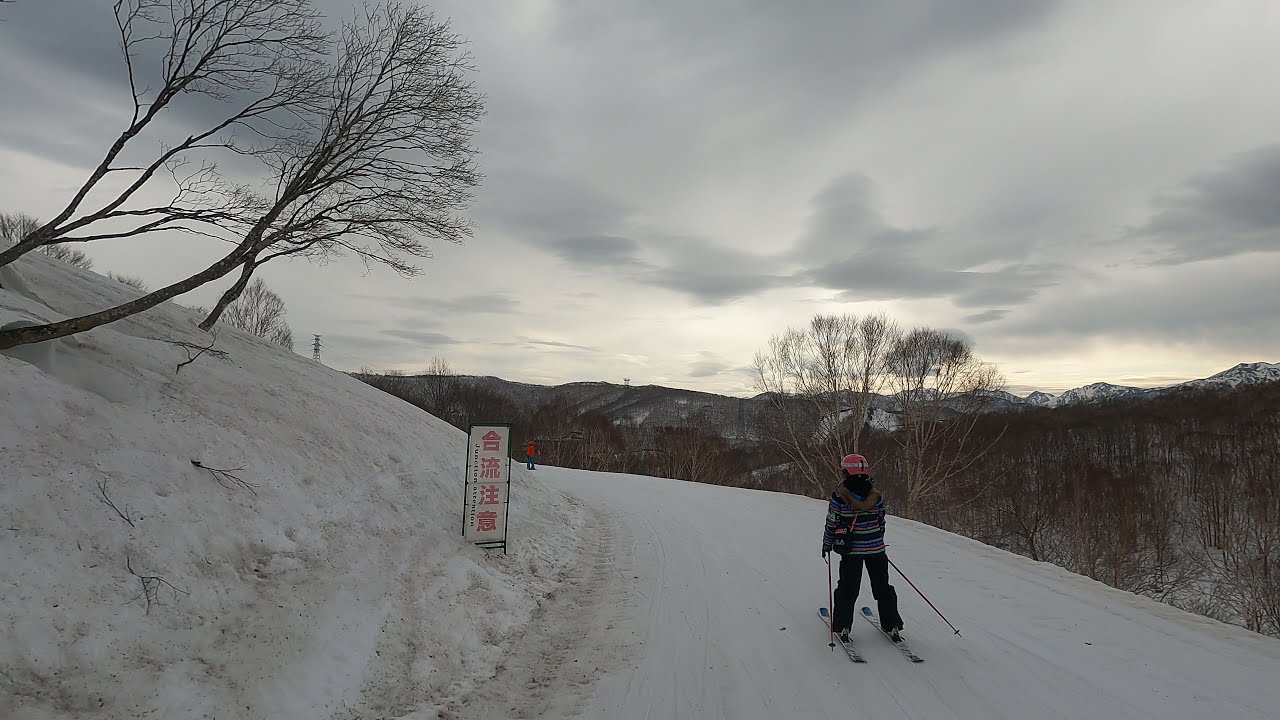The image captures a vivid outdoor scene of a young skier, possibly a teenager or in their early twenties, engaged in cross-country skiing on a snowy path. The individual is outfitted in black ski pants and a striking multicolored jacket featuring green, pink, light blue, and dark blue stripes. They are also sporting a pinkish-reddish helmet and holding ski poles in both hands. The skier is moving away from the camera, which appears to be a freeze-frame from a GoPro video, providing a view from a helmet perspective. 

To the left of the skier, there is a snowy slope with several leafless trees protruding from the ground. Adjacent to the path, a white sign with red Chinese characters stands on a metal stake. The trail appears winding, disappearing around a curve. In the background, the scenery is dominated by a mountain range and more bare trees, all under a gray, overcast sky with ominous clouds attempting to part for the sun. The setting, characterized by realism, conveys a chilly and adventurous atmosphere.